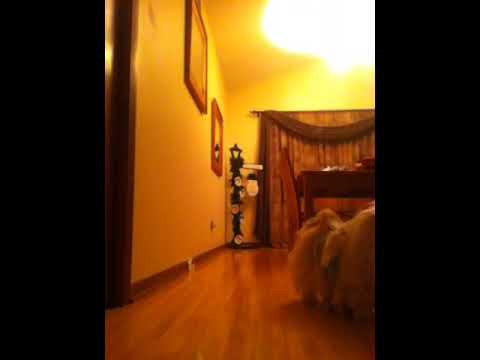The image depicts the interior of a room with a cozy, warmly-lit ambiance. It has thick black vertical borders on the left and right sides, and appears as though the photograph was taken close to floor level, showcasing shiny hardwood flooring. The walls are white but appear yellowish-orange due to the intense lighting from a bright overhead light on the ceiling. 

On the left side of the room, there is a dark brown doorframe, and further down this wall, hang two framed photographs. The rear of the room features red curtains, possibly concealing a window or door, and beneath these curtains, there is a wooden table. In the back corner, a statue resembling a street lamp adorned with festive decorations is visible, enhancing the room's homey atmosphere. On the right side of the image, a light-colored chair or a bed is partially visible, draped with what looks like a collection of fabrics or scarves almost reaching the floor. The detailed elements and warm lighting create an inviting and intimate setting.